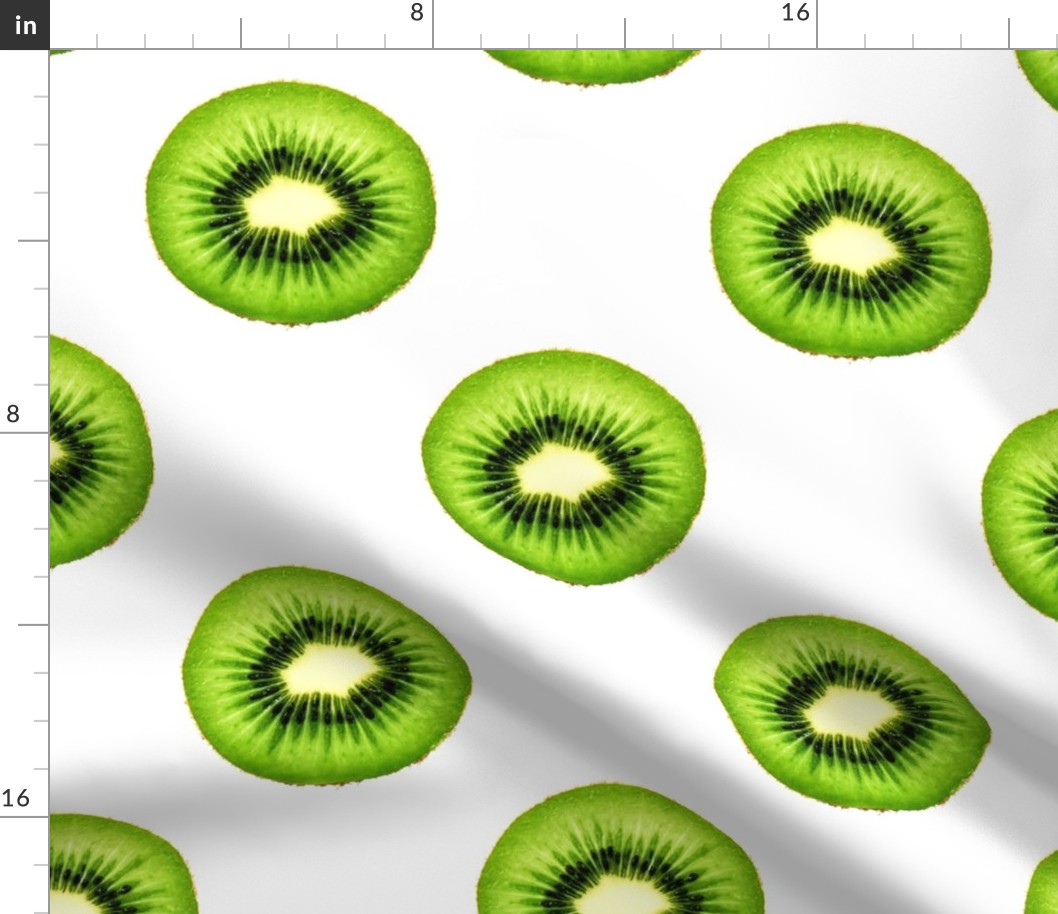The image is a detailed photograph of a white fabric or paper background that has a series of bright lime green kiwi slices arranged in a pattern. The fabric shows visible folds and creases, adding texture to the image. Each kiwi slice reveals a striking interior with a black ring of seeds surrounding a lighter, slightly yellowish-green center. The slices are evenly distributed across the fabric. A 21-inch square ruler frame borders the photograph, with measurements marked in inches along the top and left edges. Notable increments, including 8 and 16 inches, are clearly visible. The overall setup gives the appearance of a meticulously arranged product photograph, emphasizing both the kiwi slices and the structured measurement frame.